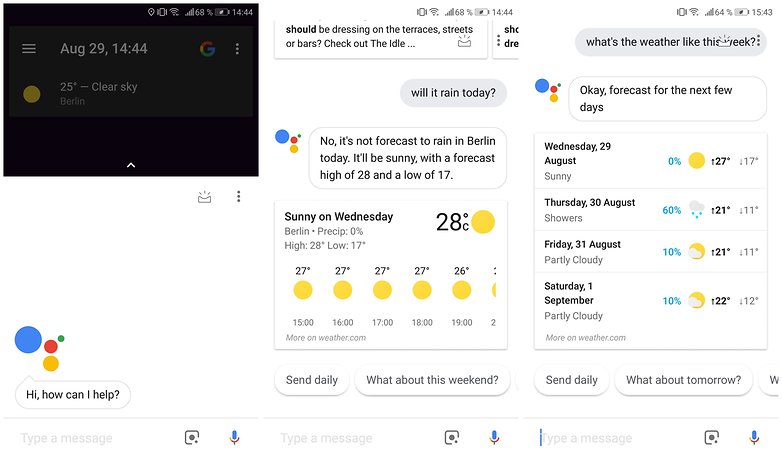This image showcases a weather website interface, featuring a dual-image display. The first image is smaller, with a black background, displaying a simple interface with a three-line hamburger menu icon next to the text "20th Nov 1444." Adjacent to this, on the right, there's a "G" icon followed by three dots.

On the left side of the page, there's a gold circle icon. Below this, the text reads "25°C - Clear sky," with additional details underneath. To the right, in a white-background section, another image is displayed with the text: "Should be dressing on the terraces street up or bars check out the idle." This message ends in an ellipsis and features an icon on the right side.

Further down, the conversation continues with "Will it rain today?" followed by the response, "No, it’s not forecast to rain in Berlin today. It will be shiny with a forecast high of 20°C and a low of 17°C." Below this informative section, a box details the weather forecast with "20°C - Sunny on Wednesday." It further breaks down hourly temperatures, ranging from 27°C at 15:00 to 26°C at 19:00.

On the right-hand side, there are forecasts for the upcoming four days, each displaying the expected weather conditions and temperatures.